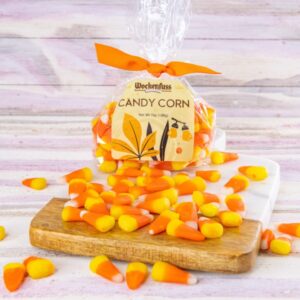The image features a clear cellophane bag of candy corn, tied at the top with an orange bow. The label on the bag reads "candy corn" and includes an illustration of an orange leaf, detailed with various shades suggesting five different kinds of leaves. The bag is placed on a square-shaped cutting board that has a visually distinct design: the front section is a light tan wood while the back section appears to be white marble. This contrast adds a striking backdrop for the candy corn, some of which has been poured out onto both sections of the board and scattered around it. The candy corn pieces are cone-shaped with a distinctive color pattern: a wide yellow base, a vibrant orange middle, and a white tip. The cutting board rests on a surface that looks like painted wood, very light gray or whitish, with visible wood grain textures. The overall setting creates a rustic yet festive ambiance, ideal for highlighting the autumnal treat.